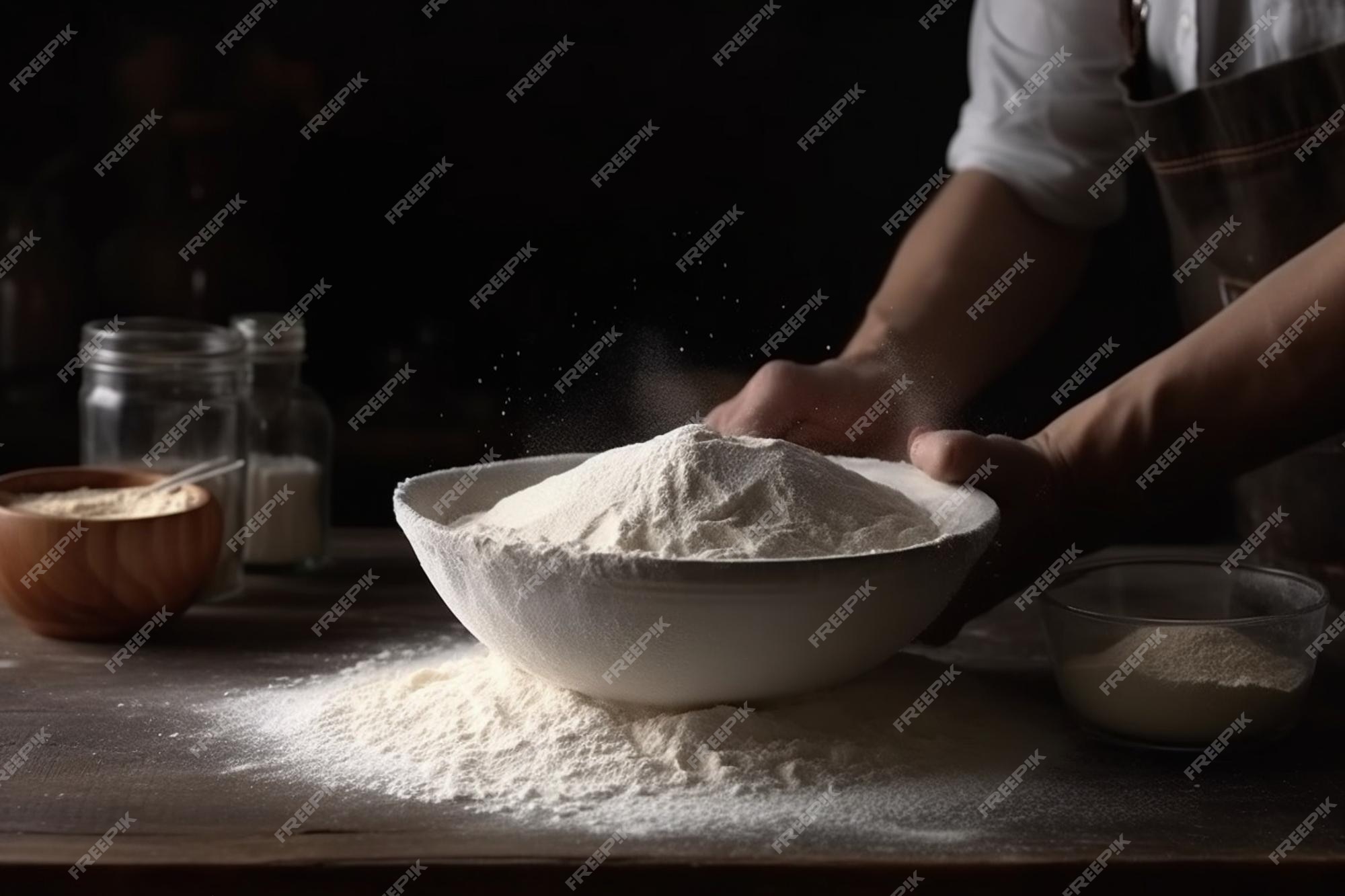In a bustling kitchen setting, a chef in a brown apron and rolled-up sleeves over a white shirt is captured in the process of baking. Central to the image, the chef holds a large, white, wide bowl filled with fine, milled flour. Some of the flour has spilled out, creating a mound on the wooden kitchen counter beneath the bowl. The scene is immersed in ingredients and tools: a smaller bowl with another flour-like substance is situated in the bottom right corner, while a wooden bowl filled with a similar powdery substance rests in the middle left, accompanied by a couple of mason jars nearby. The chef's forward-leaning posture and both hands gripping the bowl suggest an active involvement in sifting or mixing the flour, essential for the baking task ahead. This image, watermarked with "Freep K!", portrays a moment of culinary preparation, laden with scattered flour and other baking essentials.